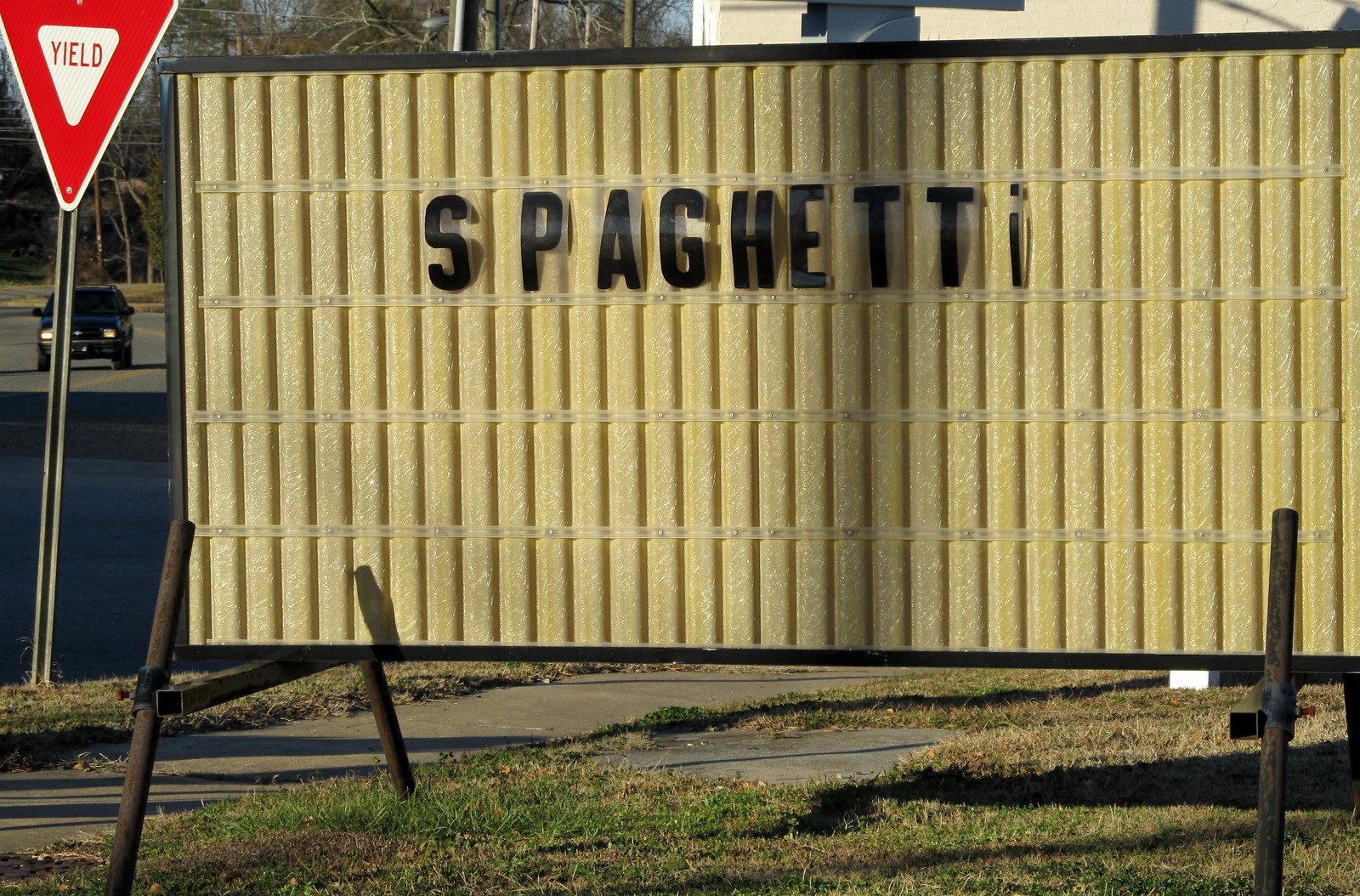In this daytime photograph, a standalone marquee with low metal legs and a plastic structure prominently occupies the forefront, displaying the word "Spaghetti" in insertable black letters on its upper half. The marquee sits on a grassy patch adjacent to a sidewalk. To its left, a metal post with a yield sign is visible. In the background, behind the yield sign, there is an SUV approaching with its headlights on. A distinct shadow bisects the marquee, running vertically through the first "T" in "Spaghetti."